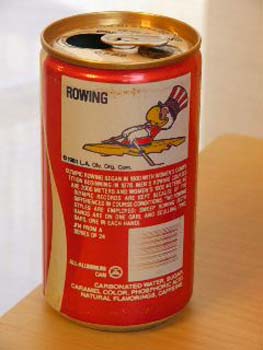This image showcases the back of a Coca-Cola soft drink can, predominantly red in color. The iconic Coca-Cola logo is partially visible on the left-hand side of the can, marked by a distinctive silver wavy line. The can rests on a light brown counter, set against a plain white background. Notably, the can has been opened, with its copper-colored top featuring the open hole.

At the top of the can's backside, a rectangular section displays a design with a white or silver background. In the upper left of this section, the word "ROWING" is printed in capital letters. Adjacent to this, there is a cartoon image of a duck engaged in rowing. The duck is depicted leaning back, with its head tilted towards the upper right corner of the rectangle. Wearing a hat with red and white vertical stripes, the duck is positioned in a gold-colored kayak. Its large, rounded beak is bright yellow. The back of the can also includes fine print in white writing and a barcode set against a silver background. Reflections can be seen on the metallic surface, adding a touch of realism to the image.